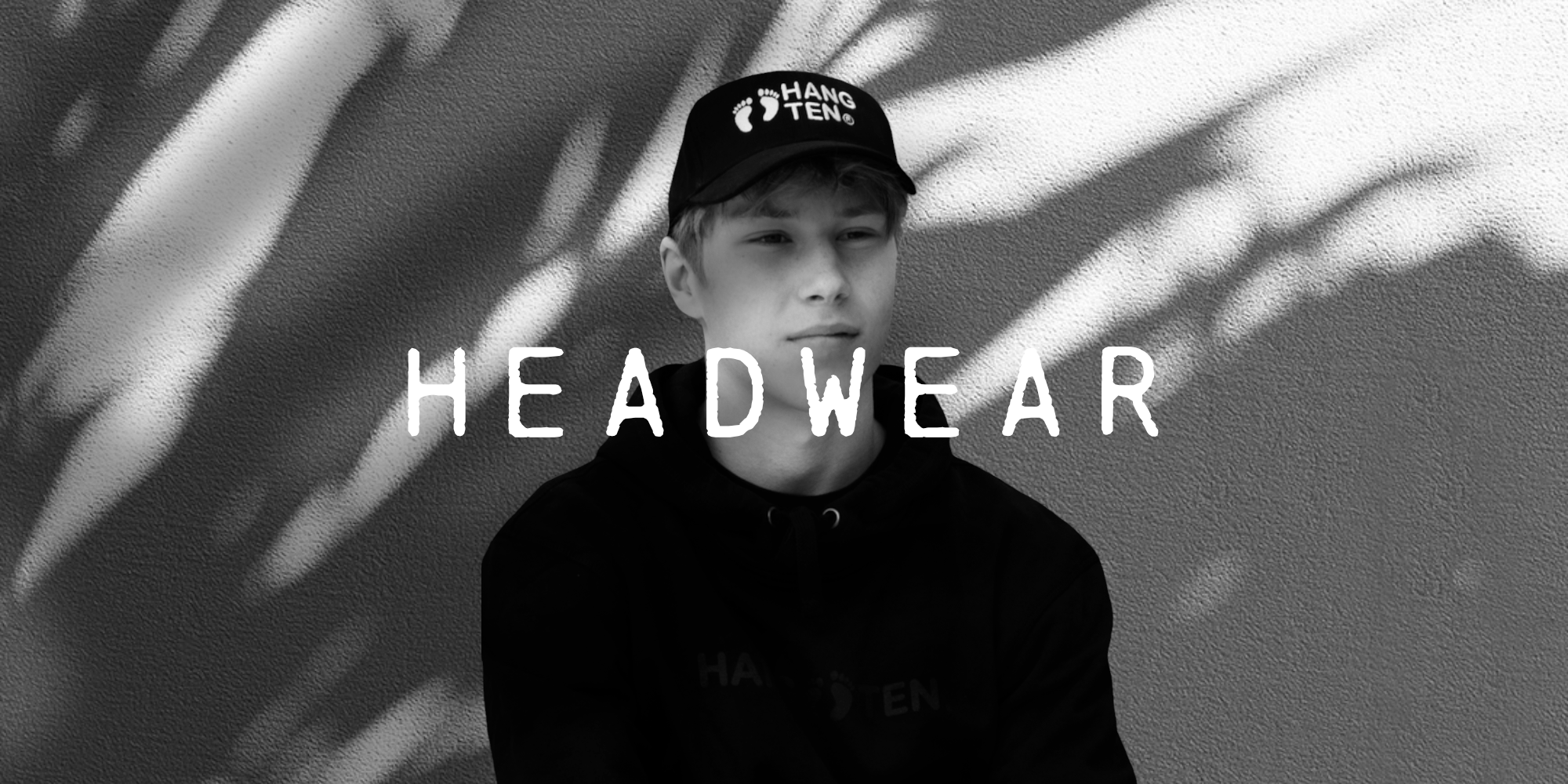The black-and-white promotional photograph is a narrow, horizontal shot featuring a young man, likely in his late teens, with a slim build and bleached or blonde hair. He is centrally positioned, looking slightly to the right with a neutral expression. The young man is dressed in a black hoodie and a black billed baseball cap that prominently displays white text reading "HANG 10," alongside two white bare feet silhouettes and a trademark icon. The cap text "HANG" appears on the first line, and "10" on the second. Superimposed over the lower part of his image, in all caps and white sans-serif font, is the word "HEADWEAR." The background consists of an abstract, out-of-focus marbled pattern in dark gray and white. Dimples are visible on either side of his nose, adding to the detailed portrayal of his youthful features. The shadowy backdrop may also include indistinct shapes that resemble branches or cloth.